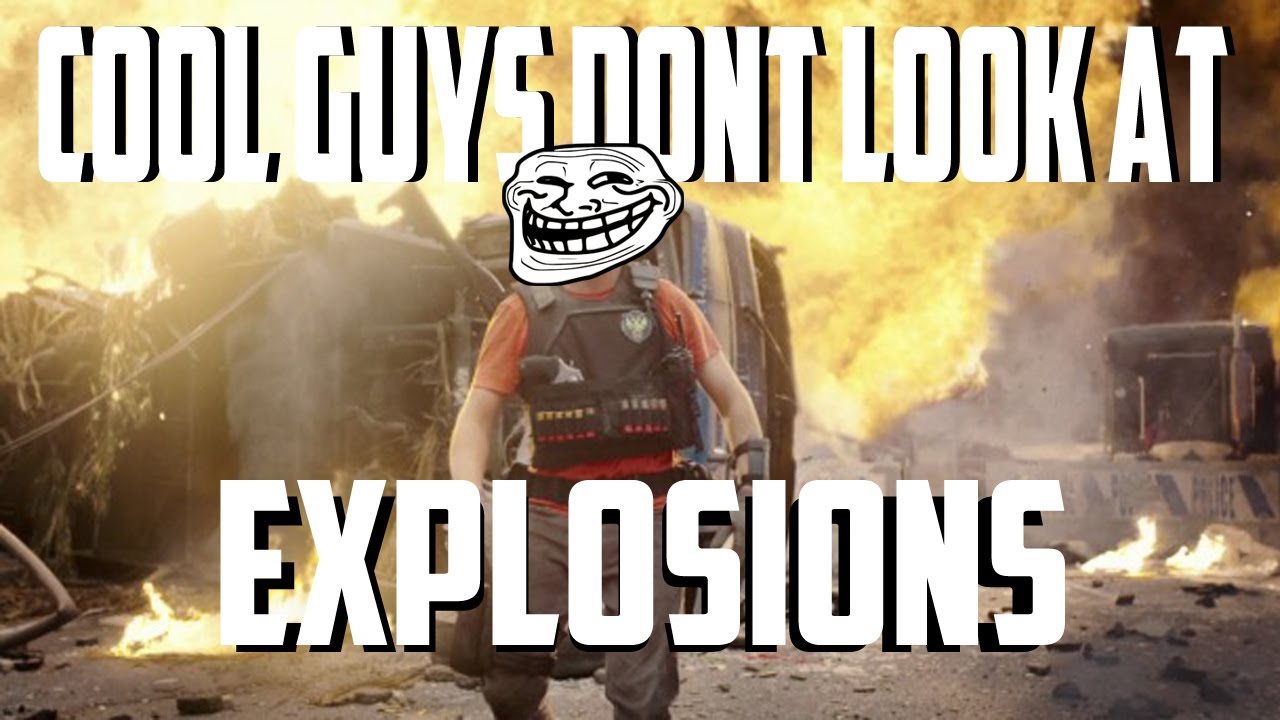In this meme-style image, there is a central figure of a man wearing a tactical vest, a red t-shirt, a gun, some ammo, a badge, and a walkie-talkie. His face is humorously replaced with a troll face, a cartoonish black and white drawing of a bald man with a squinty expression and a wide, toothy grin. The scene is set against a backdrop of chaos and destruction, featuring flipped-over vehicles and large, fiery explosions with vibrant shades of yellow, orange, and red. The destruction includes scattered objects caused by the blast. The image is captioned with large white text with a black shadow, reading "Cool guys don't look at explosions," emphasizing the man's nonchalant demeanor as he strides away from the fiery wreckage. This humorous and dramatic setup is typical of meme culture, designed to be shared on social media.